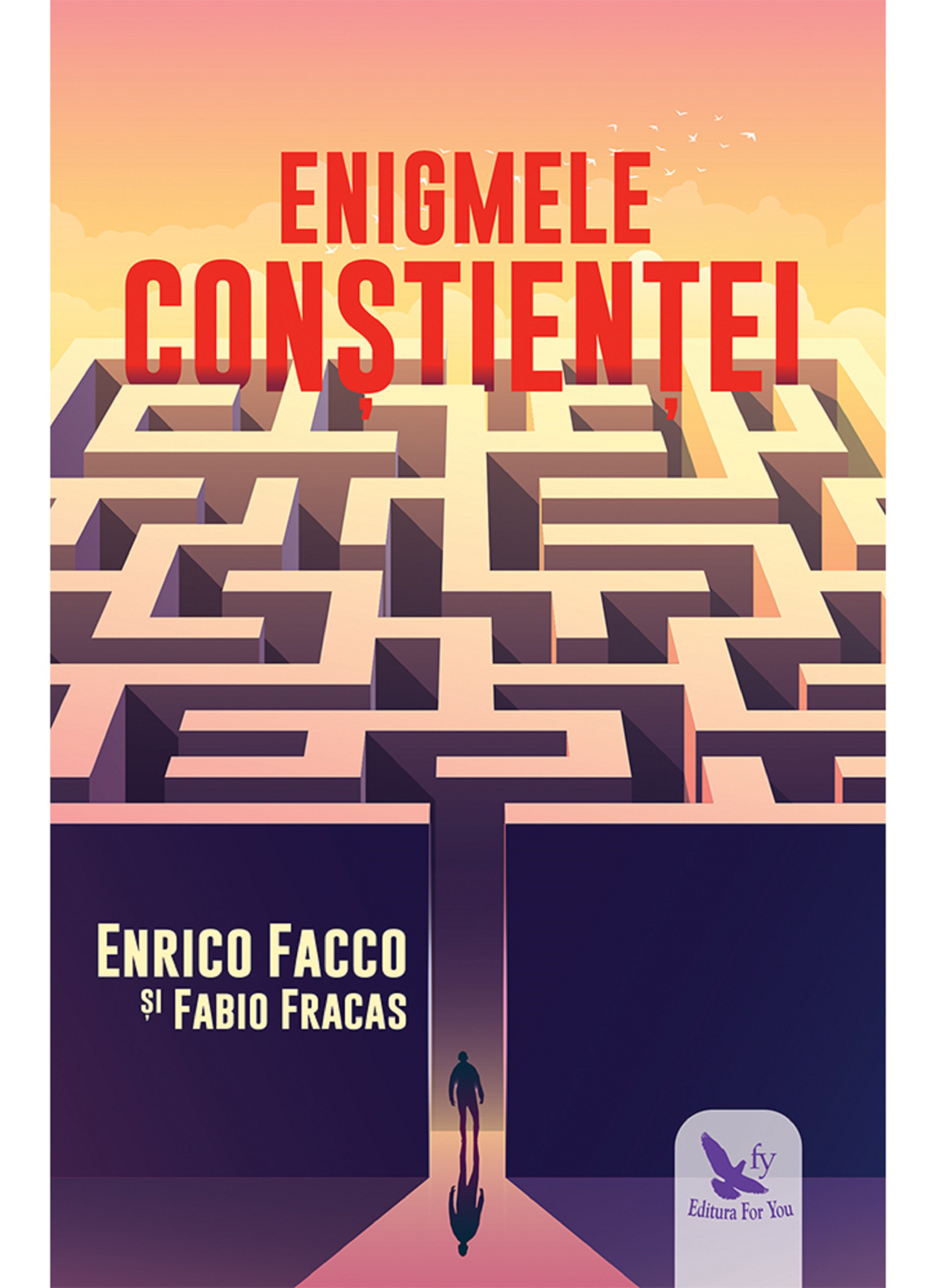The image appears to be the cover of a book, featuring a detailed and vibrant scene. Dominating the picture is a 3D labyrinth or maze with purple walls and a narrow entrance where the silhouette of a man stands, poised to enter. Above the maze, a beautiful sky transitions from orange and pink hues to a lighter beige color, dotted with white birds and soft clouds. Two lines of text in bold red capitals are positioned at the top, reading "ENIGMELE" on the first line and "CONSTIENTE" on the second. On the left side, near the bottom, the authors' names, Enrico Facco and Fabio Fracas, are written in yellow text. In the bottom right corner, there is a purple emblem featuring a flying bird and the phrase "Editora for You," alongside the letters "FY." The scene as a whole conveys a sense of mystery and adventure, inviting the viewer to imagine the journey within the labyrinth.